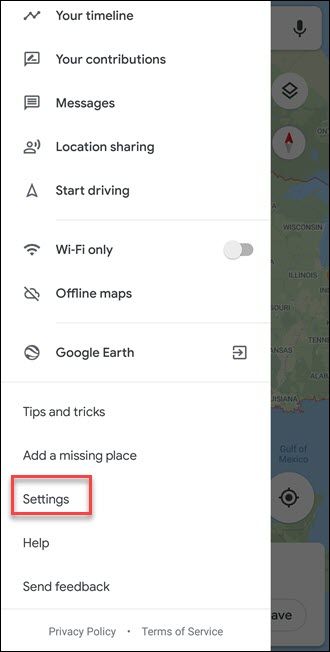This image is a detailed screenshot from a smartphone displaying the Google Maps application. The background features a partially transparent green landscape with darker green patches and white areas. On the far right side of the screen, there is a black microphone icon. Below it is a white circle containing a black square overlaid on a gray square. Next to this is a compass with a red pointer at the top and a gray pointer at the bottom.

The menu on the left side features several options:

1. "Your timeline" with a gray line graph icon.
2. "Your contributions" represented by a square with two lines.
3. "Messages" indicated by a chat bubble icon.
4. "Location sharing" signified by a silhouette of a person with two outward-curving lines.
5. "Start driving" shown with an arrow icon.
6. "Wi-Fi only" beside which there is a toggle switch set to the left; the switch is black with a gray circle.
7. "Offline maps" represented by a cloud with a line through it.
8. "Google Earth," next to an icon featuring a circle with lines resembling the Earth. Nearby, there is a square with an arrow pointing inward to the right.

Following these, there is "Tips and tricks," "Add a missing place," and "Settings" highlighted with a black color and a red square around it. Next is "Help" and "Send feedback."

At the bottom center of the menu, in gray text, it says "Privacy policy," followed by a period, and then "Terms of service."